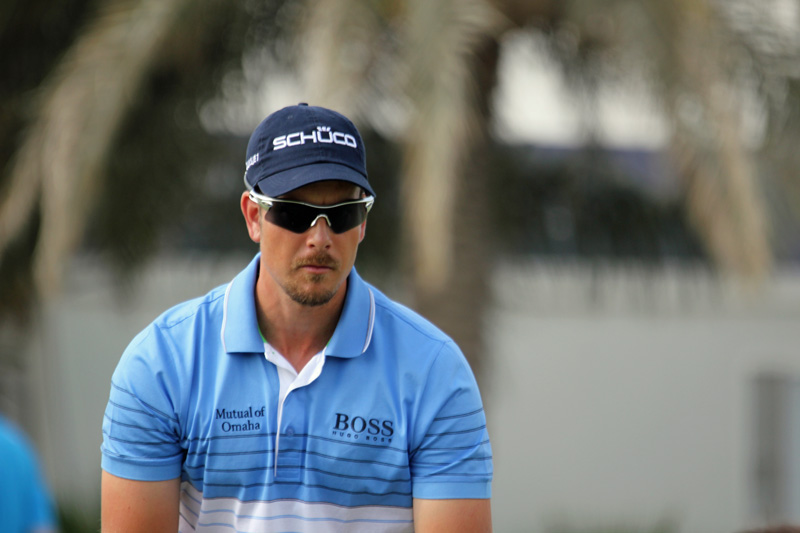In the photograph, a gentleman is seated slightly to the left of the center, set against a hazy backdrop featuring a building that appears to be a church, complete with visible support beams extending from various sides. He is dressed in a baby blue polo shirt with distinctive features: the right chest displays the acronym B.O.S.S. in black letters, while the left chest bears the logo of Mutual of Omaha in smaller blue lettering. The polo shirt features several horizontal blue stripes near the top transitioning to white fabric with additional blue stripes. The gentleman is also wearing dark aviator-style sunglasses and a blue baseball cap with white lettering spelling out C-H-O-O-C-O above the bill. He sports a very slight beard on his chin, completing his casual yet coordinated look.